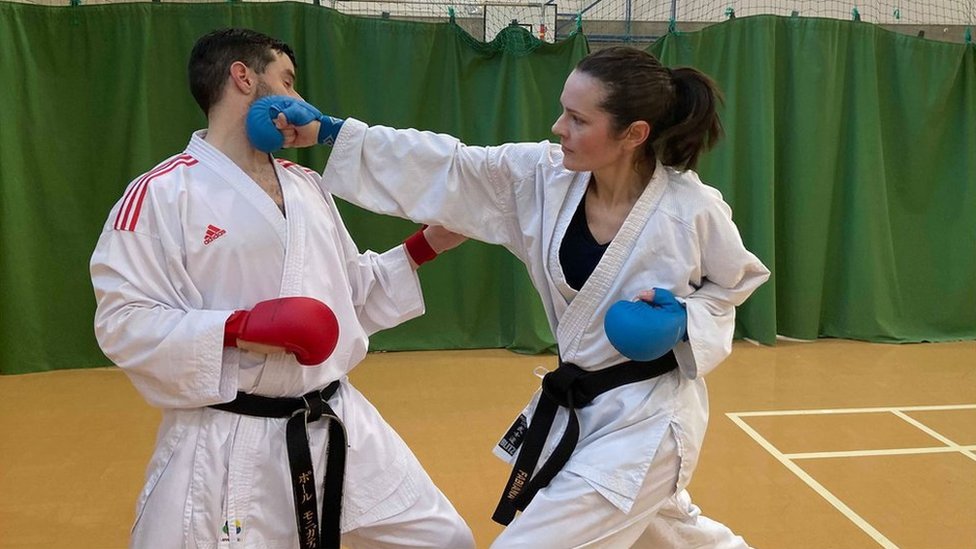In this detailed action shot, two individuals engage in martial arts practice in a gym. The woman, positioned on the right, sports dark brown hair tied in a ponytail and wears a white gi with a black belt. Underneath her gi, she wears a black shirt and dons blue fingerless gloves. She is executing a precise punch to the man’s cheek with her right hand. The man, standing on the left, has short dark hair and short facial hair. He is also attired in a white gi with black belt, which features red Adidas stripes on the shoulders and a red emblem above the right breast. He wears red fingerless gloves and his head is turned towards the left, impacted by her punch. They appear to be training on a tan-floored area with white markings, possibly a former basketball court. A green curtain stretches across the background, providing them privacy as they practice.